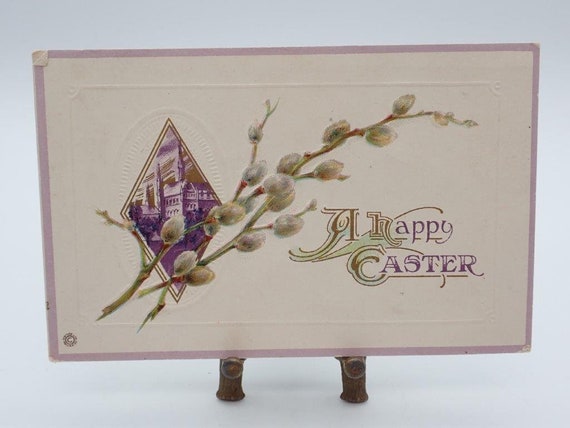The image depicts a beautifully designed greeting card or postcard set against a pristine white background, possibly displayed on a white table. The card itself is propped up by two small, wooden stands. It features a light blue frame transitioning into a faint purple border, enclosing a white interior with intricate details. The center of the card showcases a hexagon-shaped pattern combined with a diamond structure, within which a purple building is illustrated against a backdrop of a purple, white, and tan sky. Accompanying this illustration are stems with green and yellow olives, artistically painted to mimic a natural growth across the card. Adding to the elegant design, the bottom right-hand corner presents the warm message, "A Happy Easter," in purple text. Additionally, the card has white indentations that add texture to its surface, and a subtle shadow beneath the stands, giving it a slightly three-dimensional effect.